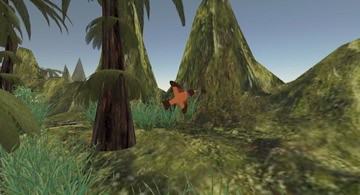The image appears to be a digitally created scene, reminiscent of a prehistoric environment or a poorly rendered video game. The landscape features various elevations with multiple hills and a flat, green grassy terrain sporadically dotted with individual blades of grass. In the far background, there are very tall, upright green and gray mountains, with some that are distinctly pointy. The sky is a solid light blue. An array of trees is present, including palm trees and one with a brown triangular trunk adorned with skirting leaves. These trees appear oddly shaped and unrealistic. A small, orange bird with black-tipped wings and a yellowish beak is seen flying in the middle of the scene. Additionally, a couple of light green bushes are scattered throughout the image.